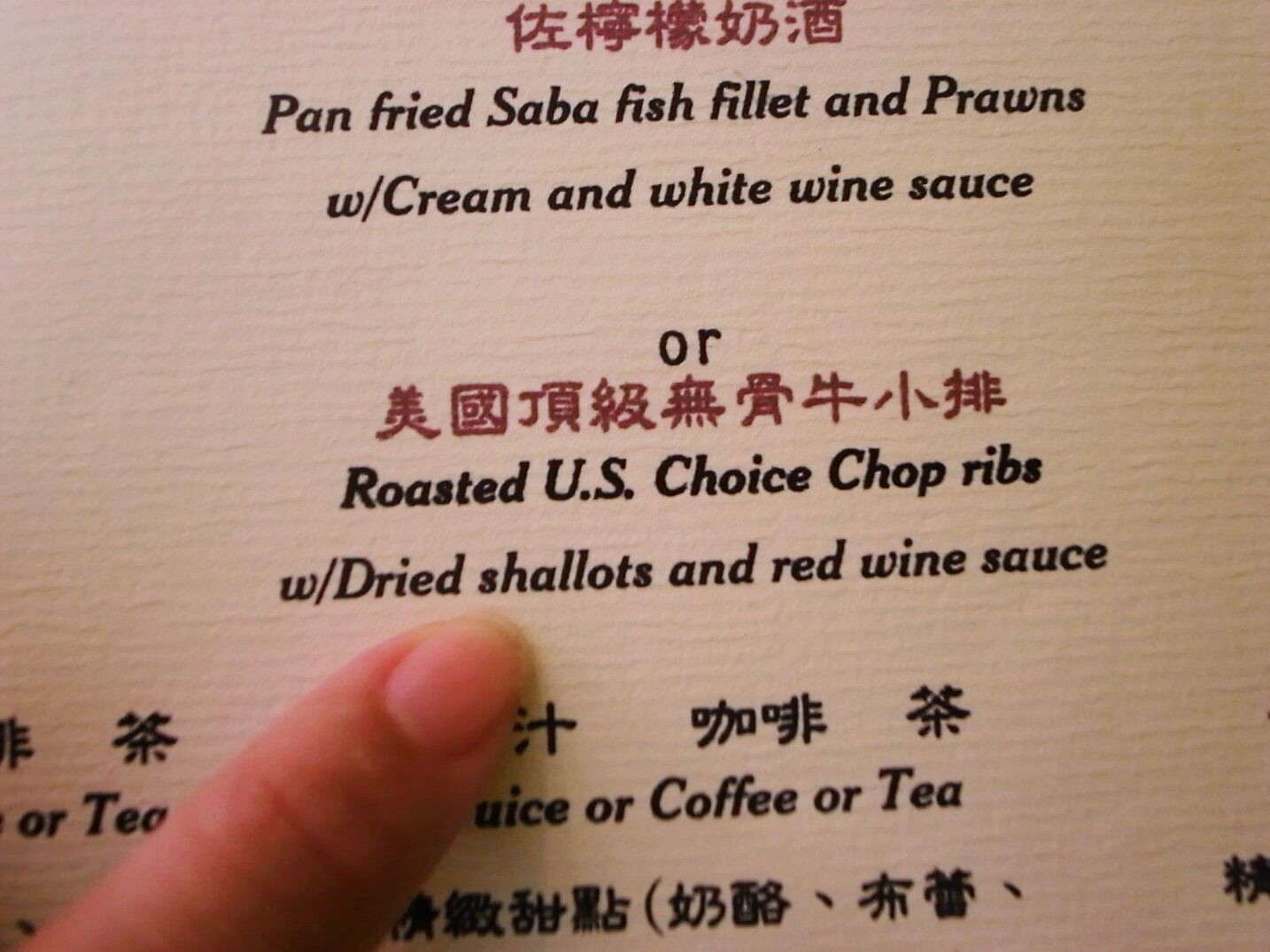A close-up photograph captures a finger pointing at a menu, emerging from the bottom left corner and extending towards the center. Though slightly blurry, the finger does not detract from the focused, textured menu, which appears to be printed on thick watercolor-type paper. The image has a slight off-white tint, likely due to soft or artificial lighting. The menu text, presented in English and an Asian language using both black and red ink, details the offerings. At the top, it lists "Pan-fried Saba Fish Fillet and Prawns with Cream and White Wine Sauce" followed by "Roasted U.S. Choice Chopped Ribs with Dried Shallots and Red Wine Sauce." The finger obstructs part of the menu, but the visible sections show "Ore Tea" to the left and "Juice or Coffee or Tea" to the right. The detailed bilingual text provides a glimpse into an enticing dining experience.